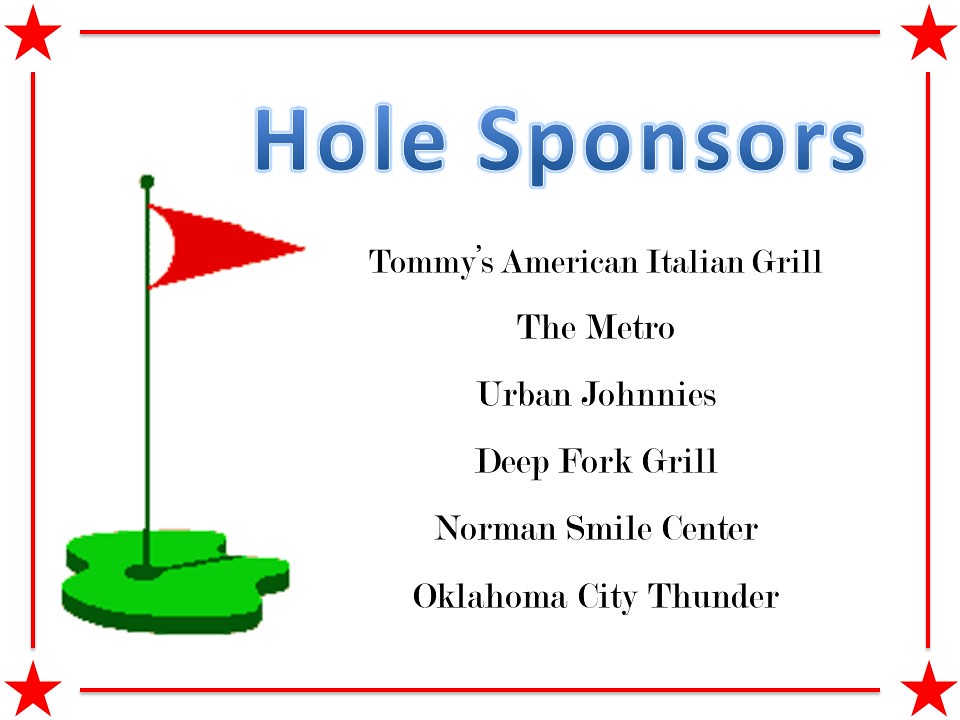This is a descriptive sign likely used on a golf course, characterized by a clean and simple design. The white square is framed by a thin red border, with a red star marking each of its four corners. The background of the sign is entirely white. The top of the sign features the words "Hole Sponsors" in large, blue letters. Below this heading, in black text, are listed the sponsoring entities: Tommy's American Italian Grill, The Metro, Urban Johnny's, Deep Fork Grill, Norman Smile Center, and Oklahoma City Thunder. On the left side of the sign, there is a digitally created image of a golf green with a flagstick. The flag is triangular and red, and it casts a noticeable shadow on the green. The detailed and straightforward layout highlights the sign’s purpose of acknowledging the sponsors for a particular golf hole, indicative of common sponsorship signage seen at golf tournaments.